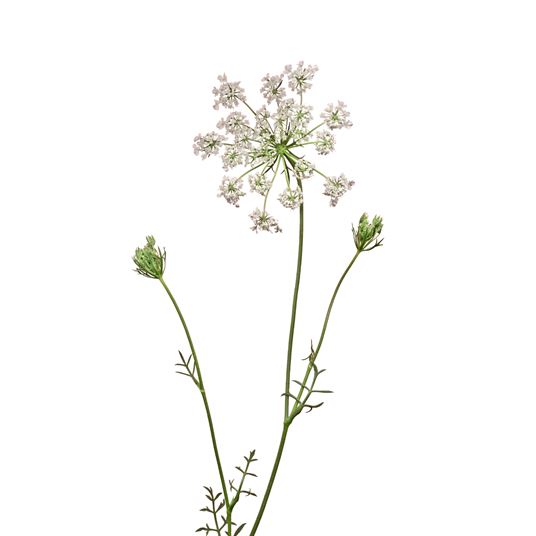The image depicts a hyper-realistic portrayal of a plant with three green stems set against a plain white background. The central stem features a striking cluster of flowers with white petals, which seem subtly tinged with a light purplish hue. The flowers in full bloom reveal centers that might be yellow or green, adding a delicate contrast to the white petals. Small, needle-like leaves adorn the stems, enhancing the botanic authenticity of the portrayal. Notably, several buds are seen on the stems, suggesting imminent blooming. One of the stems is prominently taking center stage, with an offshoot bearing another yet-to-blossom flower. The entire scene is devoid of text, focusing solely on the intricate details and natural beauty of the plant life.